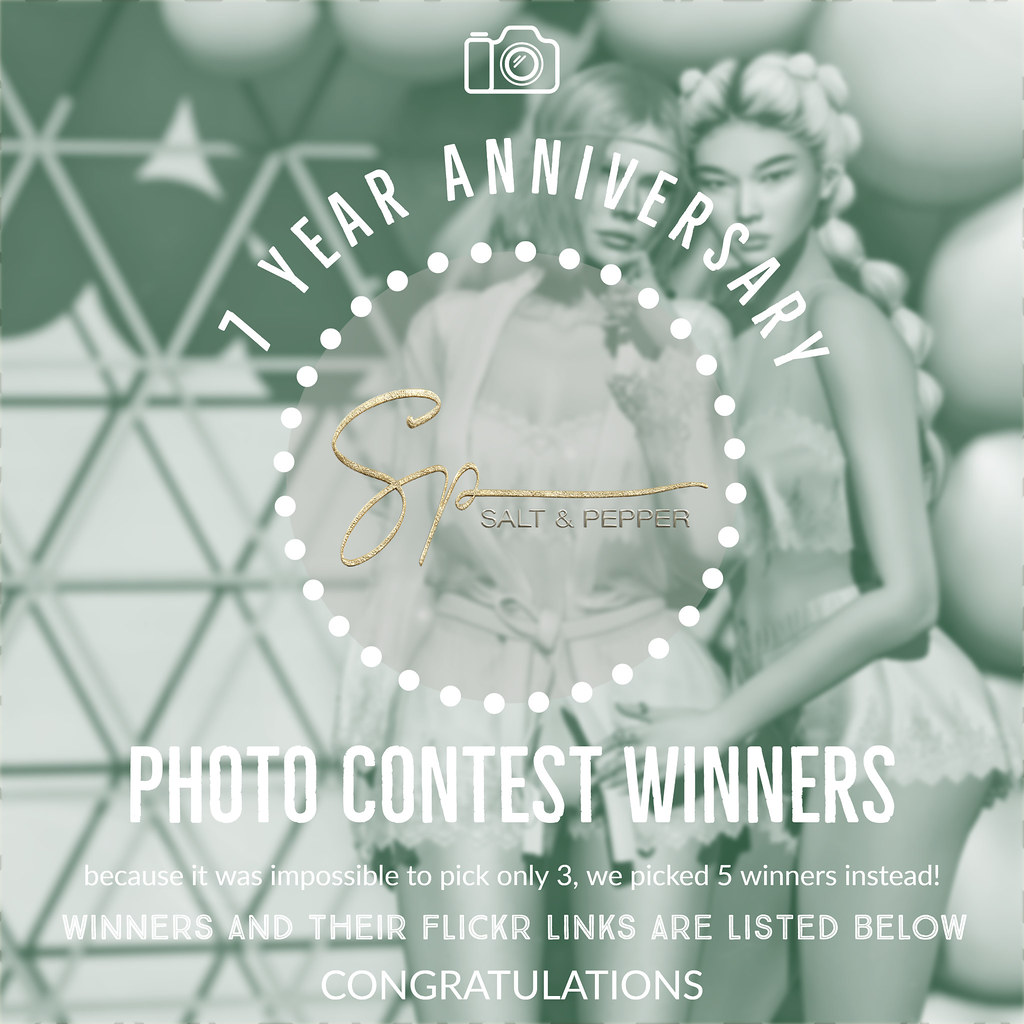The image features a black-and-white photograph of two women standing close together on the right side. One woman, appearing Japanese and dressed in skimpy lingerie, places her hand on the thigh of the second woman, who has short hair, is Caucasian, and wears pajamas-like lingerie. They’re posing in front of a fence, adding a touch of intimacy to the scene. 

Overlaying the photograph is promotional text indicating it's the "Seven Year Anniversary" for "Salt and Pepper" (SP), highlighted within a circle of white dots. Each word - "seven-year anniversary" and "SP" - is styled in white text. At the top of the overlay, there’s an icon resembling a camera. Underneath this, and within the dotted circle, it announces, "photo contest winners" and details that, since it was impossible to select only three entries, five winners were chosen. The message concludes with "Winners and their Flickr links are listed below. Congratulations!" 

This comprehensive caption consolidates all repetitive and significant elements from the three descriptions, giving clear attention to shared details and image specifics.